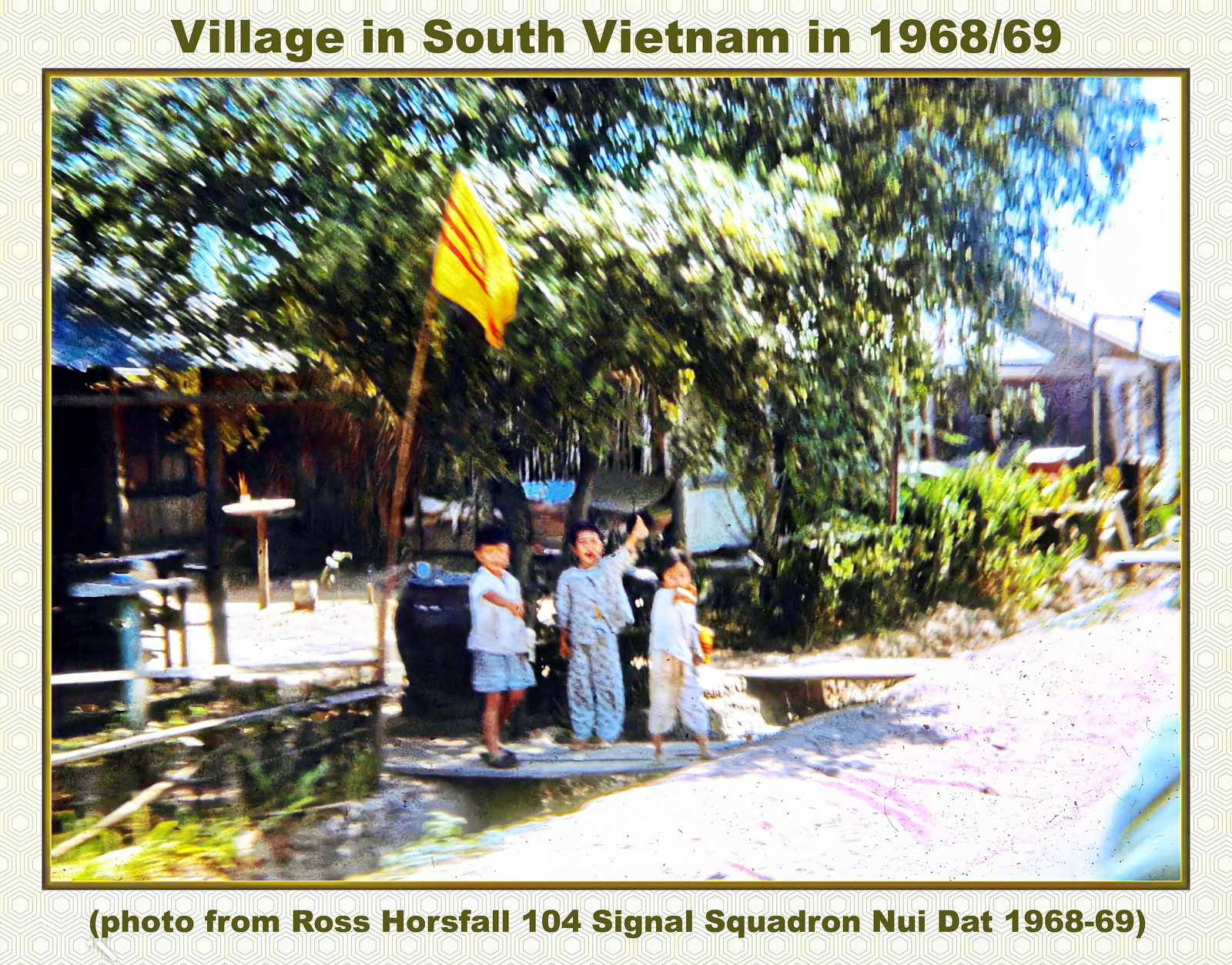The image, titled "Village in South Vietnam, 1968-69," shows a daytime outdoor scene with three children standing on wooden planks near a small house. They are dressed in white and blue clothing, resembling pajamas. Behind them, a lush backdrop of green trees and bushes adds to the vibrant landscape. A yellow and red flag flutters from a flagpole on the left side of the image. The children, standing next to a roadway or driveway area, appear slightly blurry, suggesting movement either from them or the photographer. The image is framed with a dark green border. At the bottom, a footnote in brackets reads, "Photo from Ross Horsfall, 104 Signal Squadron, Nui Dat, 1968-69." The scene is brightly lit by natural sunlight, enhancing the details of the blue sky, the foliage, and the small rural structures that include water tanks, fencing, and stools.